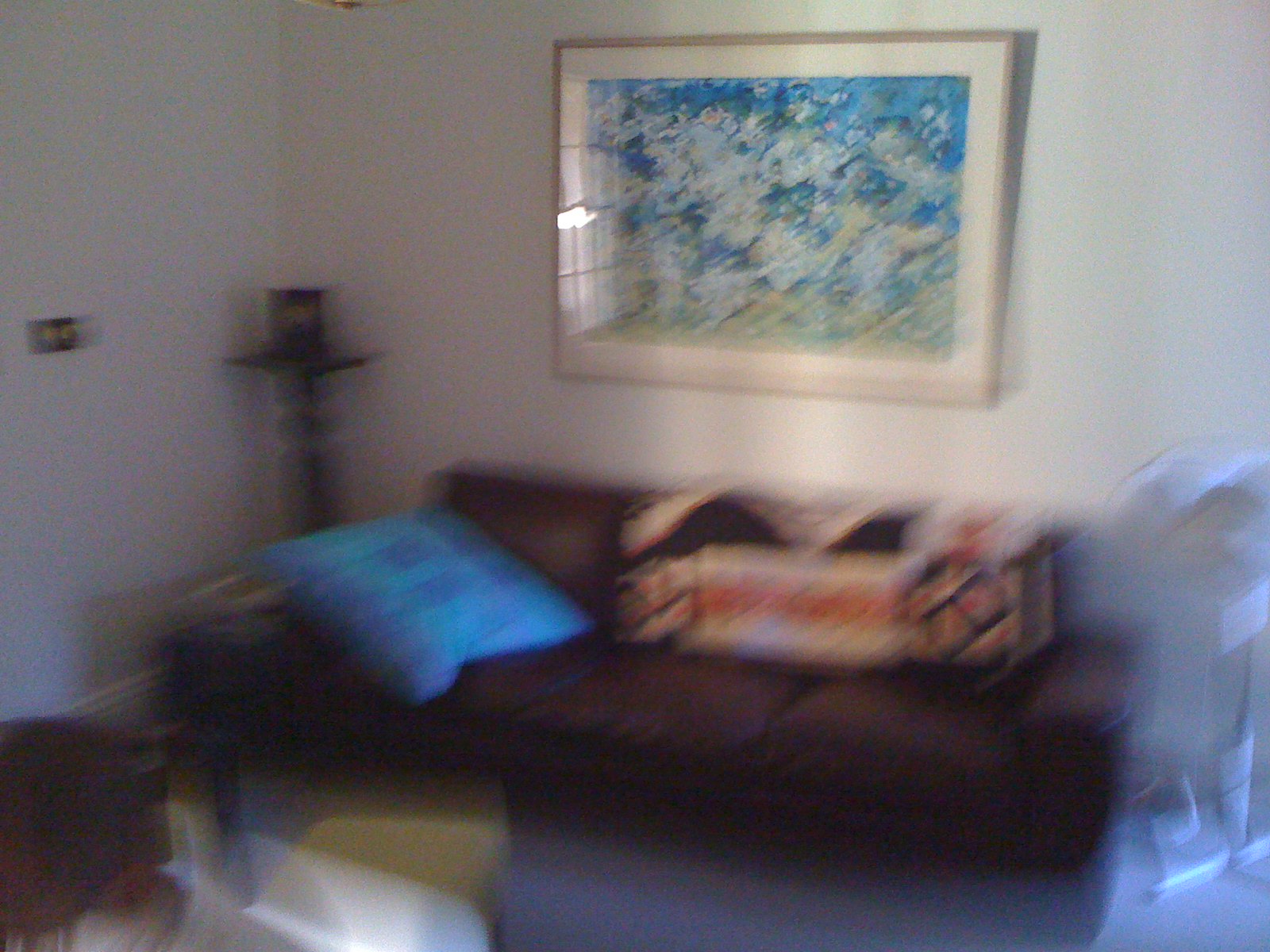In this somewhat blurry image of a living space, the general layout and key features are still discernible. The back wall and the back left wall are both painted white. A tall, black nightstand with a spindle-style design and a flat black top stands prominently in the scene. Atop the nightstand sits a purple vase. Positioned against the back wall is a brown sofa, adorned with a blue pillow and draped with a white, red, and black mosaic-style blanket. To the right of the sofa stands a white plastic pedestal fan. In the bottom left corner, a tan, silver, and brown swirl is visible, although its exact nature remains indeterminate.